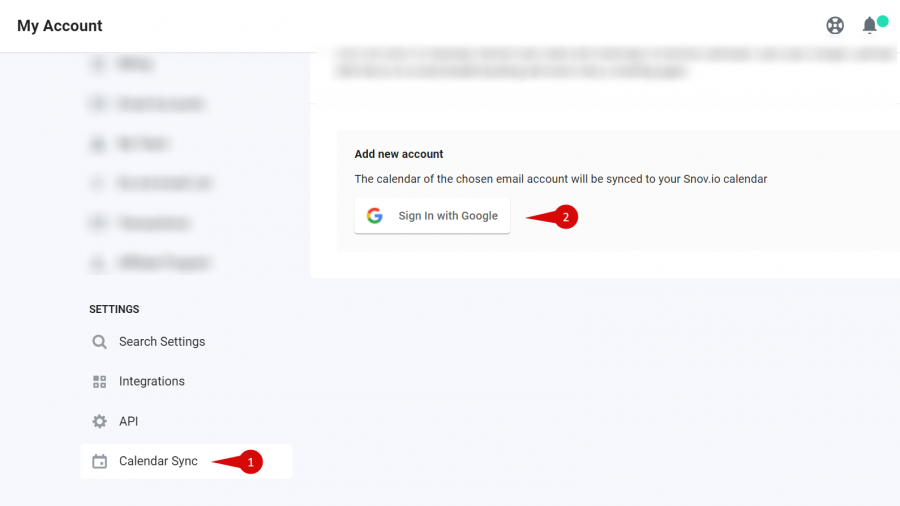Screenshot of a website interface displayed on a computer screen. The top navigation bar features "My Account". On the left-hand side, there's a vertical menu including options such as "Settings", "Search Settings", "Integrations", "API", and "Calendar Sync". The "Calendar Sync" option is highlighted with a red notification badge showing the number "1". On the right side of the interface, there is a prompt reading "Add New Account". It is followed by the message: "The calendar of the chosen email account will be sent to your calendar." The specific calendar in question is named "Snow Joe Calendar". Below this message, a button labeled "Sign in with Google" is displayed, suggesting a user action to integrate the calendar.